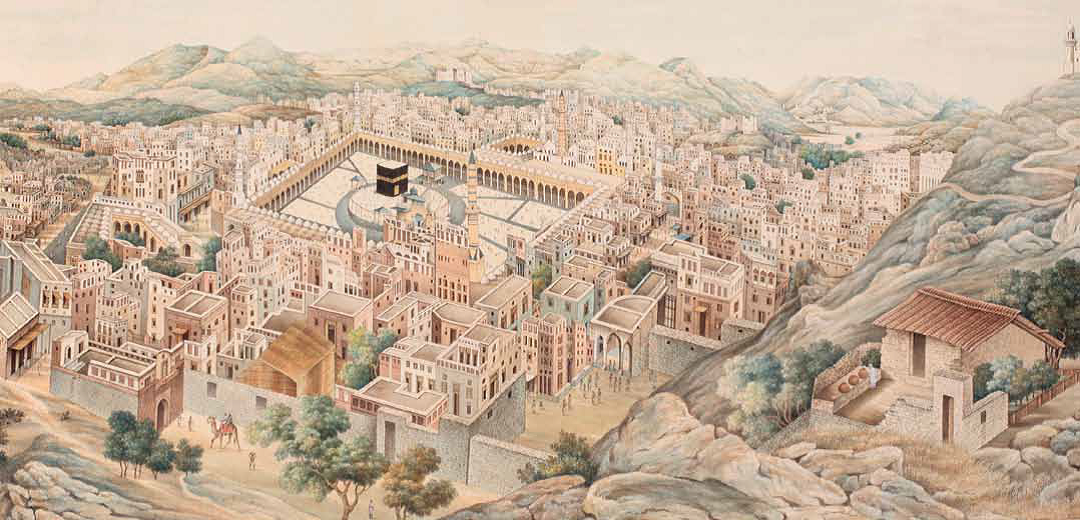This is an artist's rendering of a city nestled in a valley, encircled by mountains. Executed in muted tones of beige and brown, with green accents suggesting trees, the artwork has a slightly soft, impressionistic quality. The focal point of the city is a central plaza, featuring a stone floor and a prominent dark brown tower or perhaps a detailed fountain or statue. Surrounding this rectangular city center are numerous buildings of varying heights, many with small windows and constructed from stone. On the right-hand side, perched atop a hill, there's a notable stone house with a brown roof. To the left, a raised bridge with curved arches stretches over the cityscape. In the distance, trees and occasional splashes of greenery break up the muted coloration, adding depth to the hinterland. The composition conveys a sense of tranquility and timelessness, with small figures and cows visible in the foreground, reinforcing the serene village-like atmosphere of this sprawling urban scene.